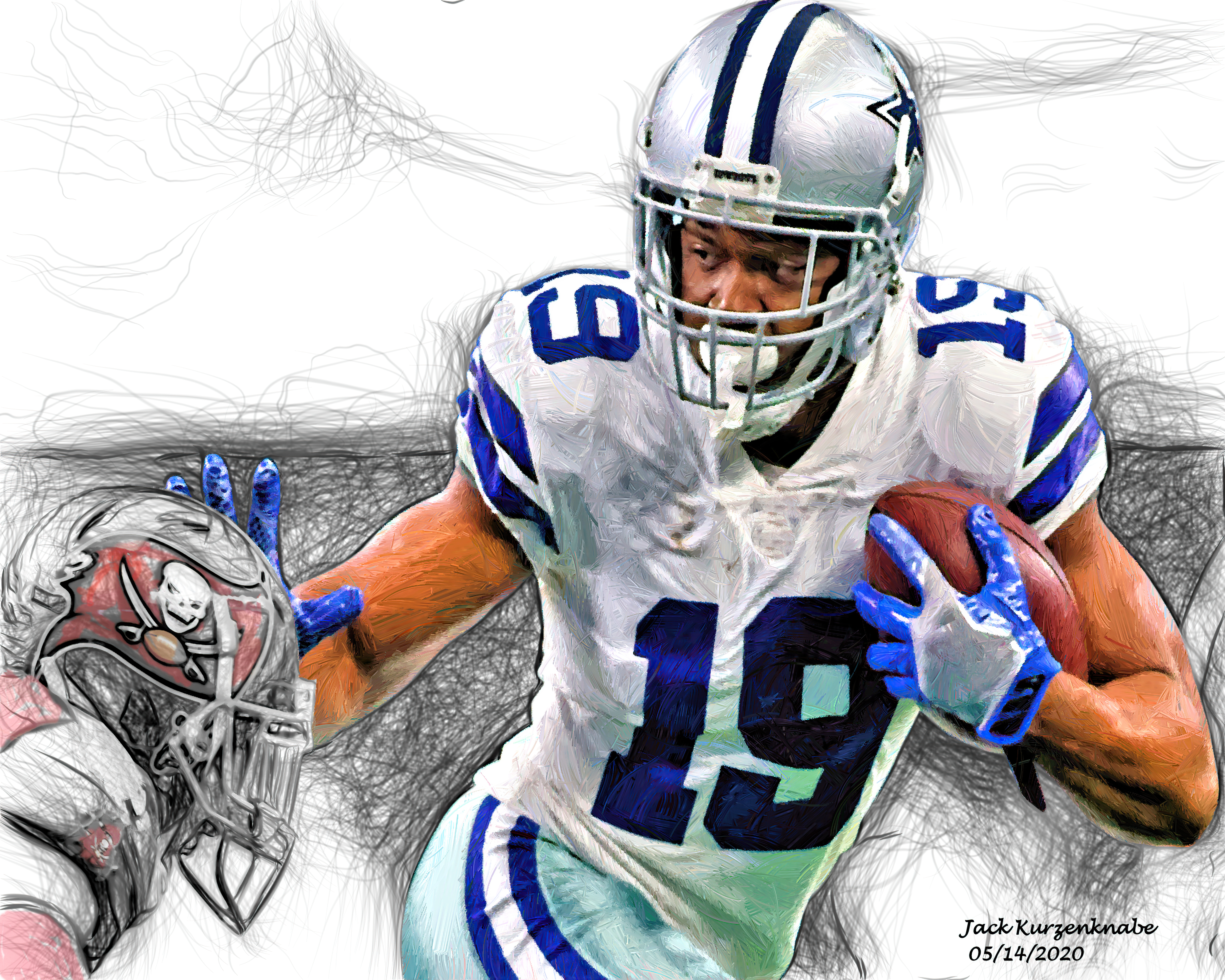The image is a stylized, almost pencil-sketched rendering of a football scene featuring a Dallas Cowboys player, wearing a white jersey with blue numbers and stripes, prominently numbered 19. He is captured mid-motion, running with the football tucked under his left arm and both blue-gloved hands raised. The player is also equipped with a Dallas Cowboys helmet, silver face mask, and a white mouth guard. In the scene, he appears to be looking towards a defender from the Tampa Bay Buccaneers, who is approaching from the side. The defender’s head and parts of his shoulder are barely visible from the bottom left, giving the impression of an imminent tackle. The dynamic portrayal emphasizes the intensity of the play, with detailed focus on the player's equipment and attire.